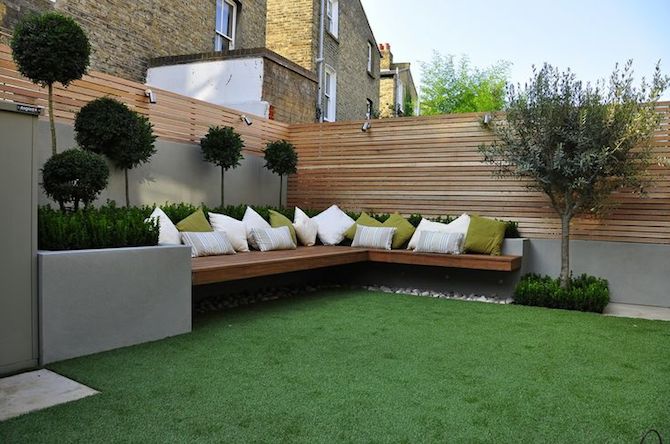The image depicts a beautifully designed, well-maintained backyard area adjacent to a house on the left side, featuring a sleek, modern appearance with brick walls and white accents on the windows. Dominating the scene is an inviting L-shaped wooden bench with a plethora of throw pillows, mostly in white and lime green shades, enhancing the cozy ambiance. The seating structure is accented with white rocks underneath, adding a decorative touch. The backyard features lush green grass, which appears so perfectly maintained that it might be artificial turf. Surrounding the seating area are planters filled with various types of shrubbery, some resembling little pom-poms on sticks, and other plants enhancing the greenery. A sturdy wooden fence with horizontal slats, approximately 12 to 15 feet tall, encloses the area. Attached to this fence are four chrome lights, providing illumination for the space. On the right side, a tree stands tall beside the bench, with additional plants around its base. The fence also features a small concrete wall at the perimeter, reinforcing the well-structured layout of this serene outdoor space.